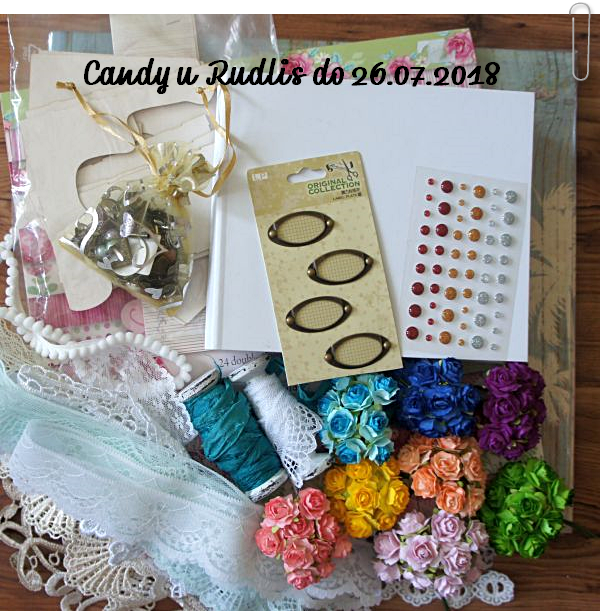This detailed photograph showcases an assortment of craft items neatly arranged on a wooden surface. At the top of the image, black cursive text reads "Candy U Redless DO 26.07.2018," possibly a label or title for the craft project. The items are spread across a wooden table, with some resting on a light blue scrapbook paper adorned with white palm trees. Among the items, there is a clear sheet of round stickers in maroon, gold, and silver varieties, varying in size. To the left, four bronze-colored clips featuring netted centers are mounted on a piece of cardstock. A collection of artificial flowers is arranged at the lower right of the image, featuring a spectrum of colors including light blue, dark blue, purple, peach, yellow, pink, and lavender. Also present are pieces of white lace trim and multiple spools of ribbon and thread in blue and white. Scattered around the scene are small decorative metal frames or clips, oval in shape, along with a mesh bag containing miscellaneous small items, and an assortment of buttons and other embellishments. The meticulous arrangement highlights the various textures and colors, providing a rich display of potential craft materials.